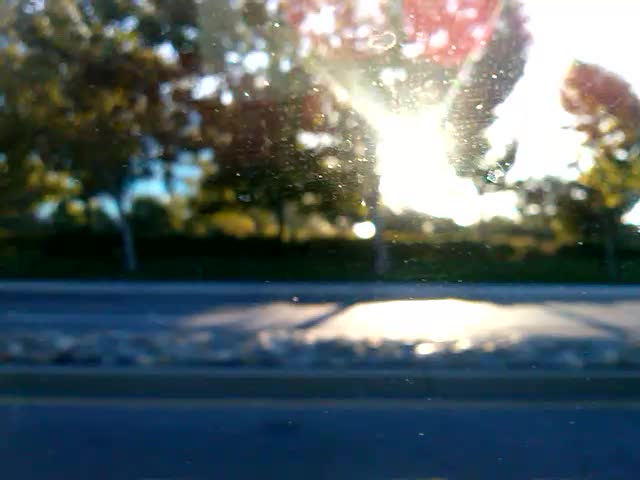The image captures a view through a glass windowpane, revealing a gray roadway divided by a green median. Beyond the median, green grass lines the sides of the road, and mature trees are visible with a mix of green foliage and patches of red leaves crowning them. The bright sun positioned centrally in the frame illuminates the ground below, creating a striking contrast and enhancing the sheen of the pavement. The dirty specks and watermarks on the windowpane are highlighted by the sunlight, appearing as grayish-white spots scattered across the glass. The scene beyond the window is somewhat blurred, obscuring finer details but showcasing the distinct silhouettes of the trees and a glaringly bright white sky in the spaces between the foliage.